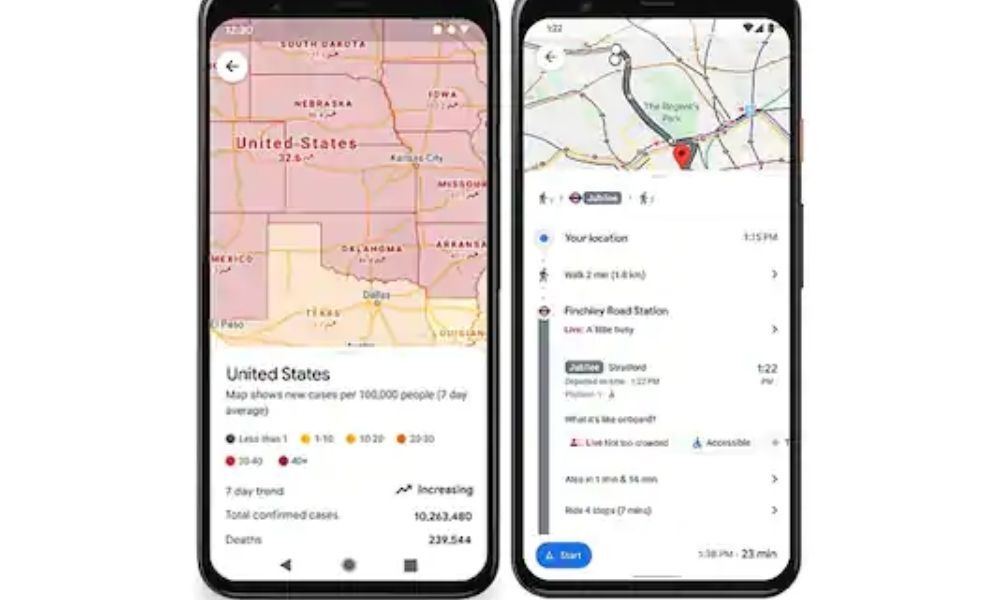This image showcases two black cell phones, each framed with a distinctive silver bar outline at the top. The phone on the left features a screen displaying a pinkish-colored map of the United States with the text "United States" aligned along Nebraska's southern border. In the top left corner of this map, there is a white circle featuring a black back arrow icon. Despite the image's blurriness, some text is discernible: a white section below the map reads "United States" in black text, and the map is described with terms like "more cases per 100,000 people" and "age." Various colored dots—black, yellow, tan, orange, red, and burgundy—are scattered across the map. Near the bottom, text reads "seven-day trend, total confirmed cases and deaths," with an emphasis on increasing trends indicated by a bold, black "increasing" text and an adjacent jagged up arrow. Large numbers like "10,262,400" are also visible, though further details are obscured.

The phone on the right shows an additional map, although its specific location remains unclear due to the image's blurriness. It contains the text "your location" and indicates directions for someone walking, represented by a small pedestrian icon on the left. It likely displays the text "Century Road Station," though this cannot be conclusively verified. A prominent oval blue button with white lettering reads "Steps" or "Start," and bolded black text at the bottom right corner indicates "23 minutes." Additionally, navigation icons—a black back arrow, a black circle, and a black square—are visible at the bottom of both phone screens.